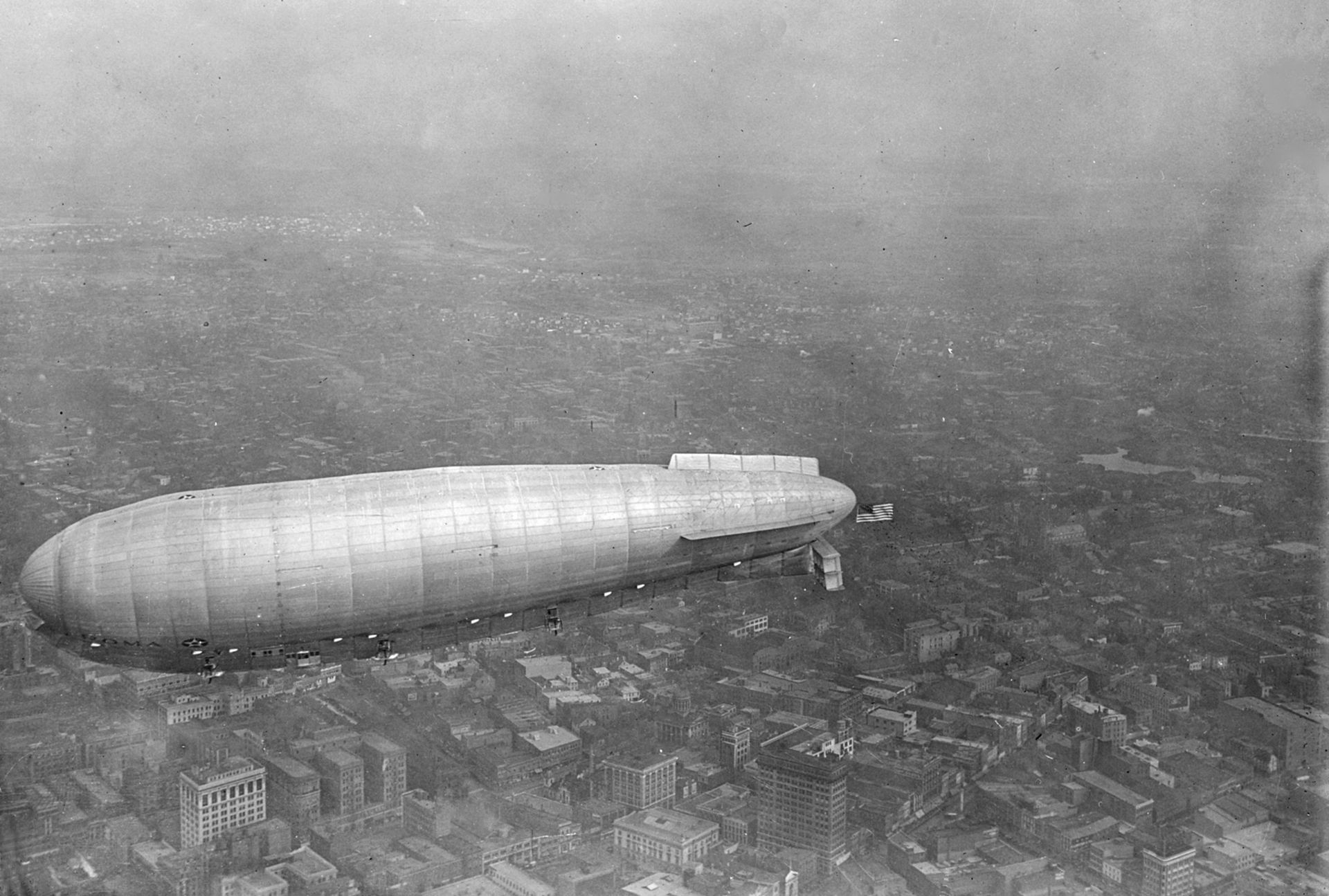This is an old-fashioned, black and white photograph capturing a massive blimp hovering over a densely packed urban area. The scene exudes a vintage aura, likely dating back to the 1920s or 1930s, an era when such technology was prominent. The blimp is positioned just under halfway up the image, slightly to the left, and extends across more than half of the frame with its elongated, silvery-gray body. A darker gray fin stretches across the bottom of the blimp, and additional fixtures seem attached to its sides, indicative of its operational requirements.

The backdrop features a sprawling cityscape, with innumerable buildings ranging in shades of gray, some shrouded in darker shadows. An American flag is draped at the far back of the image, suggesting the photograph was taken over a large American city. The scene is enveloped in a hazy, smoky atmosphere, rendering the background misty and slightly blurred, as if captured on a foggy day or due to the limitations of the photographic technology of the time. The vantage point appears elevated, possibly shot from another aircraft, enhancing the dramatic and historical essence of the image.